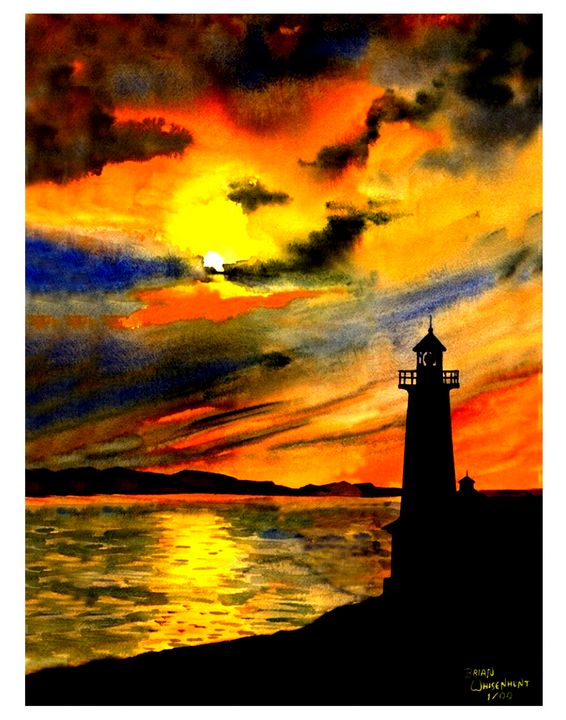This painting depicts a lighthouse silhouetted against a vibrant, fiery night sky. The tall, rectangular artwork employs highly saturated watercolors to create a dramatic scene. Positioned on the right side, the black silhouette of the lighthouse stands central in the image, overlooking a large body of water that mirrors the sky above. The land beneath the lighthouse extends from the lower right corner, curving downwards towards the bottom left. To the left of this land, the reflecting water is accented with hues of orange, blue, and green. In the distance on the horizon, faint black mountains add depth to the scene. The sky, an arresting centerpiece of the painting, is a dynamic canvas of orange, yellow, blue, and gray, with streaks of clouds that transition into a smoky black at the top. Although the text in the painting is too blurred to read, the vivid melding of colors and the tranquil yet dramatic setting evoke a sense of awe and wonder.